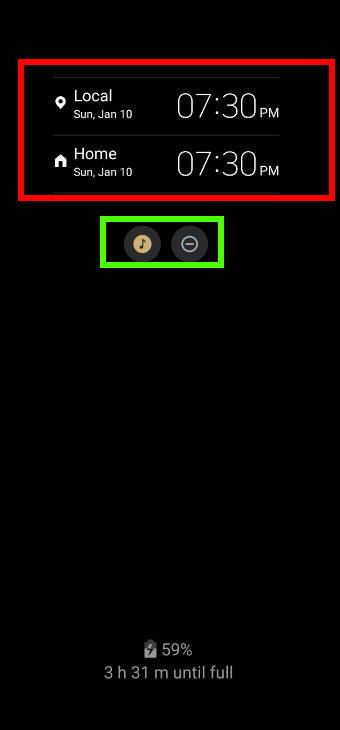The image is a screenshot from a mobile device. At the top, there are two symbols: a location icon and a home icon. Next to the location icon, it reads "Local Sunday January 10th," and to the right of that, the time is displayed as 7:30 PM. Directly underneath, it again states "Home Sunday January 10th 7:30 PM," with this section highlighted by a red box.

Below, there is a minus symbol inside a grey round button. Adjacent to this, there is another button of a similar greyish-black color, featuring a brown circle in the center with a black music note. This section is outlined in a green box.

At the bottom of the image, a battery icon indicates charging status, marked at 59% with the text "3 hours 31 minutes until full" beside it.